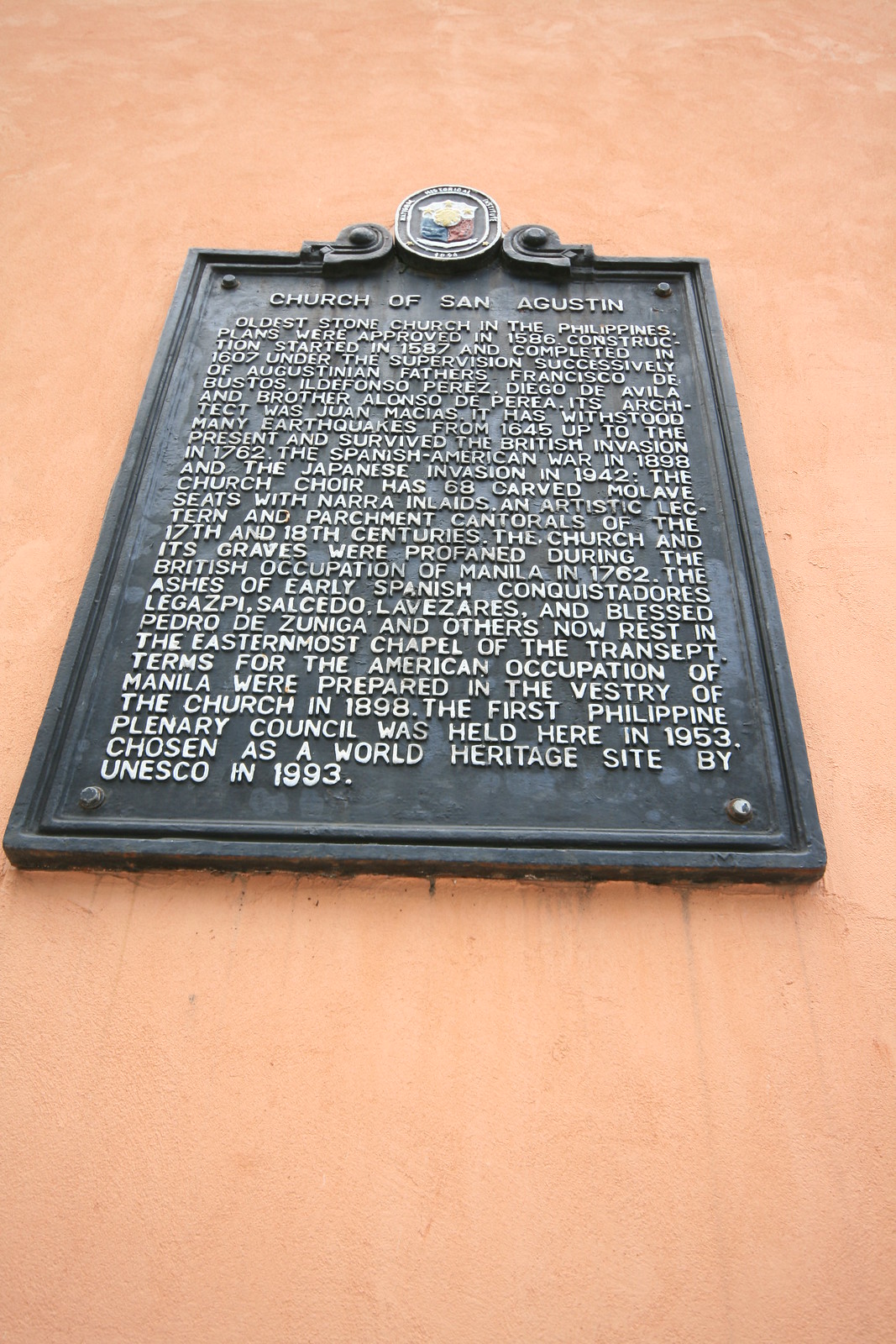This image depicts a weathered bronze plaque affixed to a terracotta-colored wall, which looks slightly pinkish-beige. The photo is taken from a low angle, making the sign appear tilted. The plaque is secured by four bolts, one in each corner, and is adorned with scroll designs at the top and a central shield-like figure that is hard to distinguish due to the distance and the sign's worn condition. The plaque, though corroded with black streaks running down the wall from its base, features embossed white lettering that reads:

**"Church of San Augustine"** - the oldest stone church in the Philippines, with its plans approved in 1586. Construction commenced in 1587 and concluded in 1607 under the meticulous supervision of the Augustinian fathers Francisco de Bustos, Ildefonso Perez, Diego de Avila, and Brother Alfonso de Pera, along with architect Juan Marcias. This resilient structure has withstood numerous earthquakes since 1645 and survived several invasions, including the British in 1762, the Spanish-American War in 1898, and the Japanese invasion of 1942. The church choir boasts 68 intricately carved mole seats with narra inlays, alongside an exquisite lectern and parchment cantoral from the 17th and 18th centuries. The graves within the church were desecrated during the British occupation of Manila in 1762, but now house the ashes of early Spanish conquistadors Legazpi, Salcedo, Lavezaris, and blessed Pedro de Zuniga, among others, in the easternmost chapel of the transept. The terms for the American occupation of Manila were negotiated in the church's vestry in 1898. Additionally, the first Philippine Plenary Council was convened here in 1953. The church was designated a UNESCO World Heritage Site in 1993.